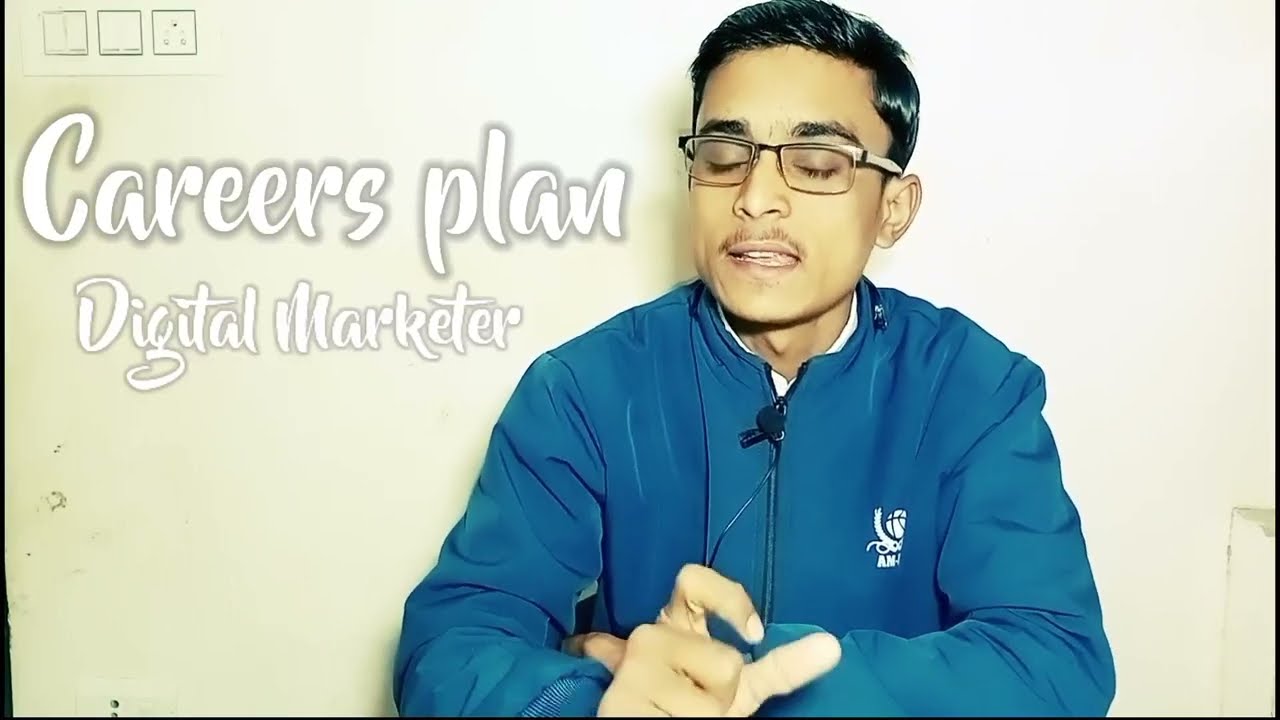In the image, we see a man positioned slightly to the right of center, sitting with both hands on a table. He is wearing a blue zip-up sweatshirt over a white shirt, with the zipper pulled up almost to the top. Attached to his shirt is a small black lapel microphone, with the cord visible and hanging downward. The man has light brown skin and short, neatly combed black hair, styled to the left, appearing glossy as if gelled. He is wearing rectangular, silver-framed glasses, and his eyes are closed, suggesting he is in mid-conversation or presentation. He appears to be explaining something, indicative of an educational or instructional setting, possibly about digital marketing. To the top left of the image, there is text in white letters stating "careers plan" and underneath it, also in white, the words "digital marketer." The colors in the image include off-white, white, gray, blue, black, tan, and pink. The background wall has a beige-greenish hue with some areas appearing slightly dirty.